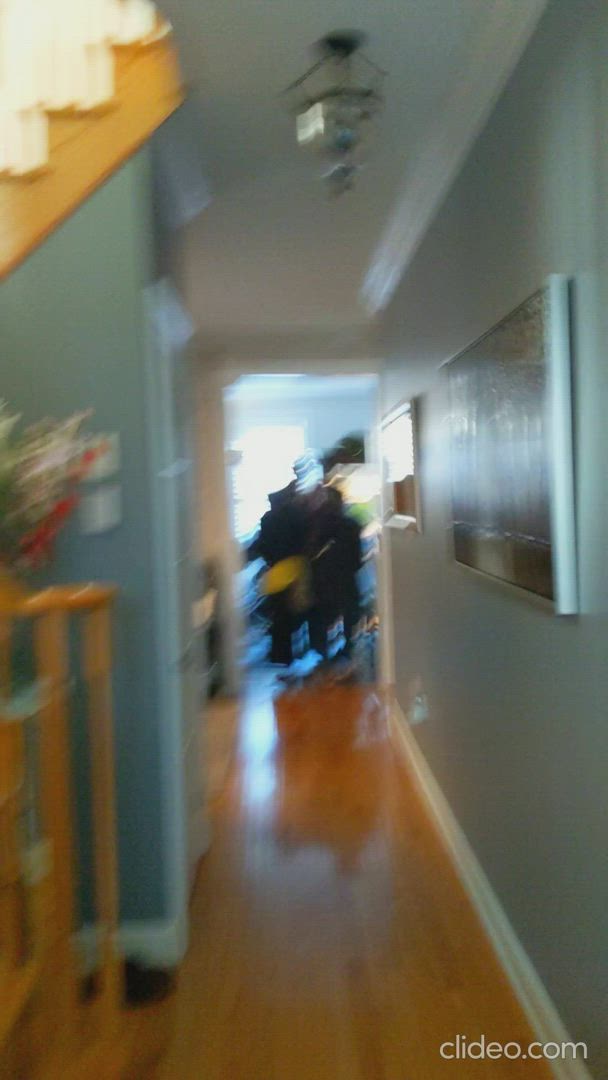A blurred photograph captures an interior view of a house, likely a hallway, characterized by a wooden floor and blue walls adorned with white trim. The apparent camera movement during the shot renders the image unfocused, offering only vague details. In the background, there is a doorway leading to another room, through which indistinct shapes suggest the presence of one or potentially two people, possibly distorted by the camera's motion. The upper left-hand corner reveals a partial view of a staircase and a tall, ornamental wooden table bearing what seems to be a floral arrangement, though the blurriness obscures specifics. Along the right-hand wall of the hallway hangs at least one framed picture, with a hint of another, although it might also be a pass-through to a different room, given the indistinct nature of the image.